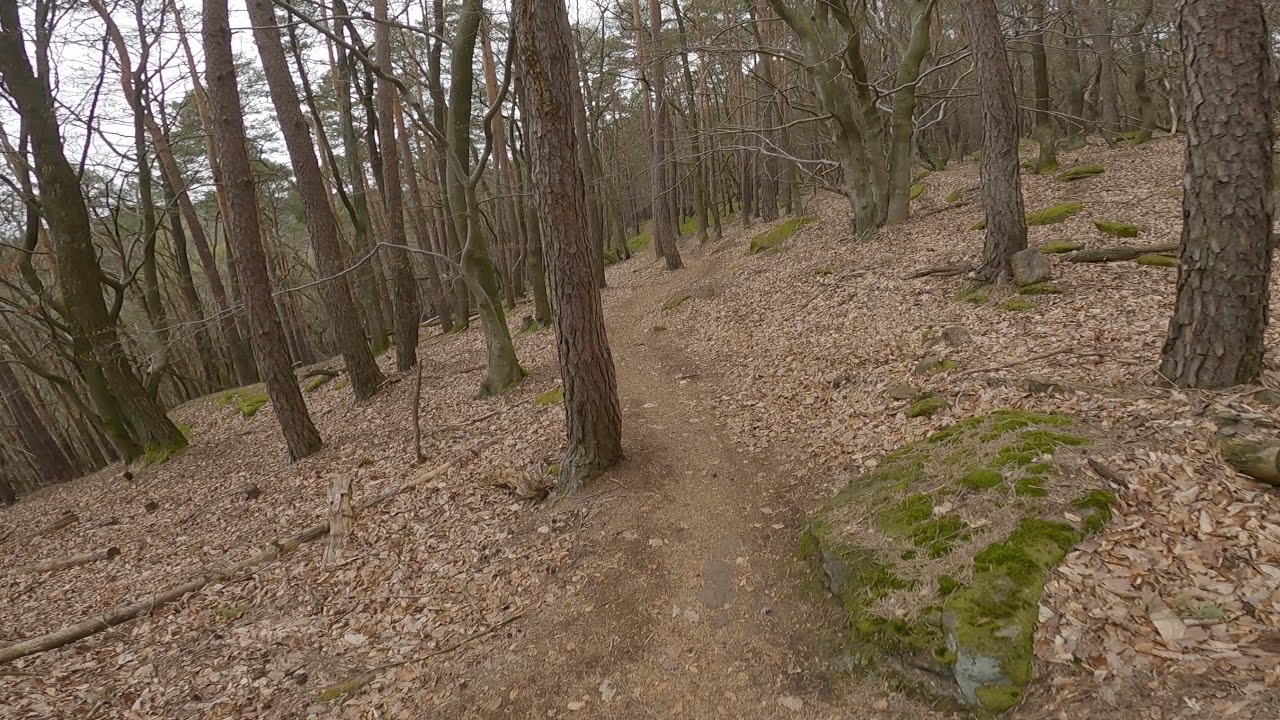The photograph depicts an overcast, possibly cloudy day in a forest during the fall or winter season. Dominated by shades of brown, the scene features a narrow, dirt path that winds slightly leftward through the trees, whose tops are cropped out of the frame. The forest floor is blanketed with brown leaves and some downed tree limbs, suggesting the accumulation of foliage over time. To the right of the path, a large rock covered in green moss stands prominently in the foreground, while the background reveals additional moss-covered rocks. The trees themselves, possibly pine, appear barren with no visible leaves, emphasizing the season. The edges of the image are cropped, focusing the viewer’s attention on the multitude of brown tree trunks stretching into the distance, and creating a serene yet somewhat desolate woodland atmosphere.